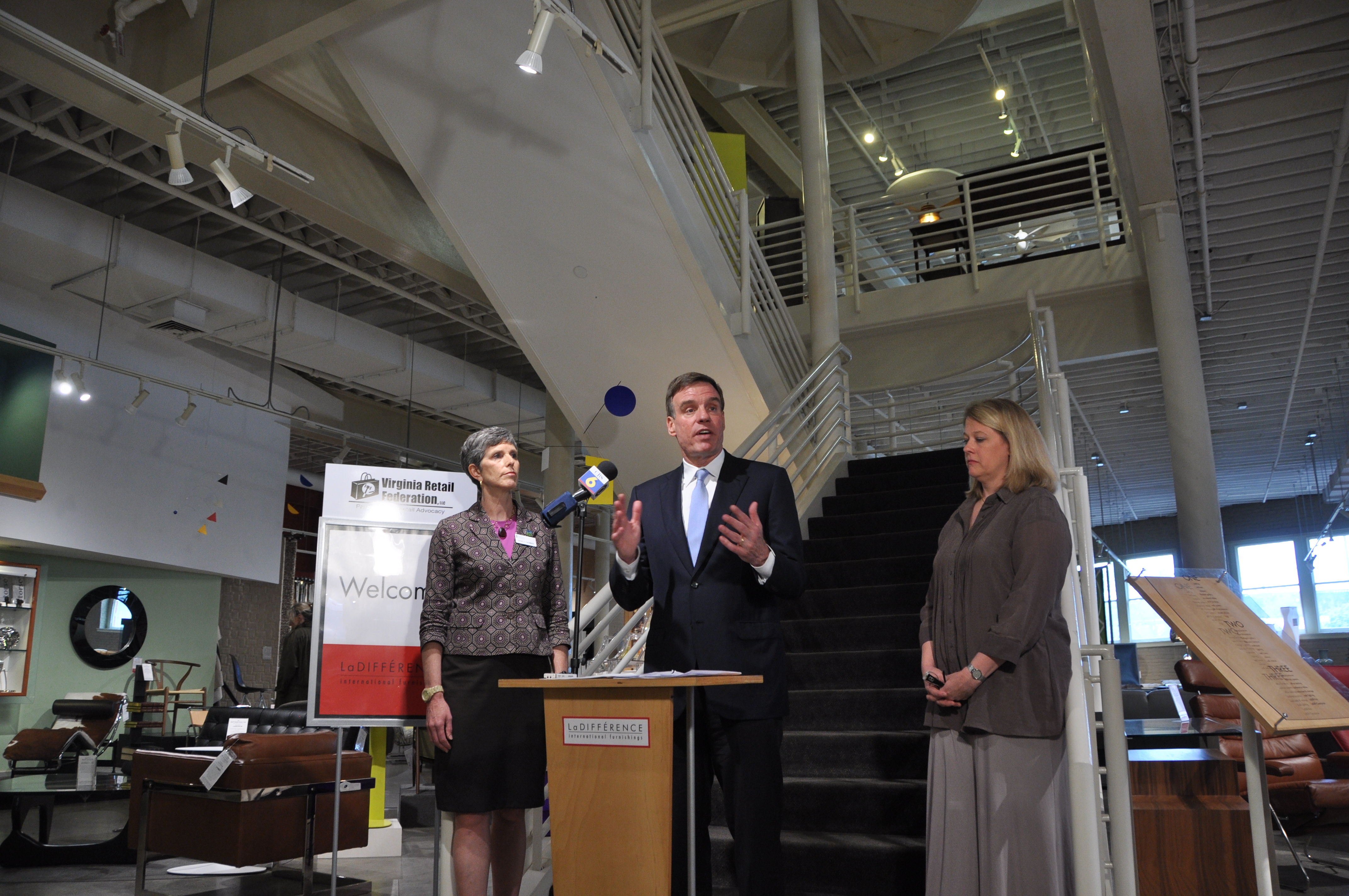In this compelling photo, a man, identified as a white male with dark hair, stands confidently at a short, brown wooden podium, which barely reaches his waist. He is dressed in a black suit complemented by a light blue tie and a white collared shirt. His expressive gesture with both hands raised suggests he is passionately delivering a speech. Mounted on the podium is a microphone marked with the number "6", indicating affiliation with Channel 6 News.

The podium features a striking white sign with a red border; the text prominently reads "Difference" with additional smaller, unreadable text below it. Flanking him are two women. On his left is a poised white female with dark and gray hair, who is dressed in a purple shirt layered with a matching gray and purple blazer, a black skirt, a name tag on her left chest, and a black necklace. She seems engaged in the moment. On his right stands another white female with short blonde hair, wearing a collared button-down gray blouse and matching gray trousers, who appears somewhat disappointed.

The photograph captures them in front of a sleek black staircase, embellished with a silver metal banister, inside a well-lit indoor venue that includes windows, hanging decorations, and desks, suggesting a formal event or conference setting.